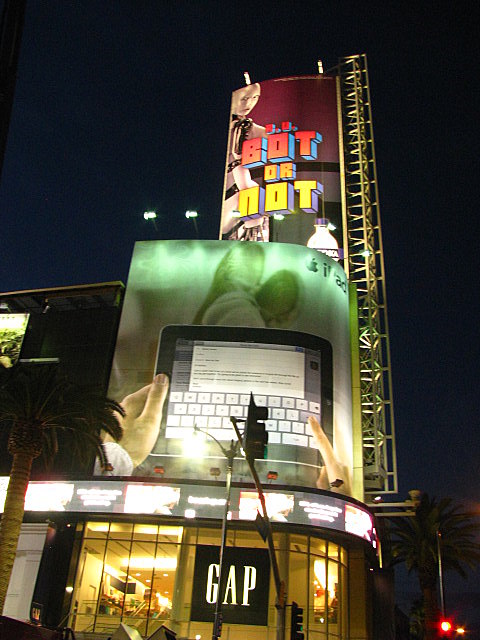**Descriptive Caption:**
A bustling nighttime scene outside the Ovation Mall in Hollywood. The sky is pitch black, with a red light faintly visible in the bottom left-hand corner, adding an eerie glow to the scene. Dominating the middle ground is a traffic light, though only its side is visible. The mall's exterior features a unique rounded edge, prominently showcasing a brightly lit Gap store on the ground floor. The store's windows glisten, and the iconic black sign with white "Gap" lettering is clearly visible. Above the Gap store, a large billboard depicts a man casually relaxing with a tablet on his lap, composing an email. His hands grip the device while his outstretched legs suggest a relaxed posture. On the left side of the building, construction scaffolding ascends upward, reaching a second billboard at the top. This top billboard features a robotic figure with the question "Are you bot or not?" in striking red and yellow text. Two additional lights are positioned to the right of this billboard. The overall ambiance is set against the stark contrast of the dark night sky.